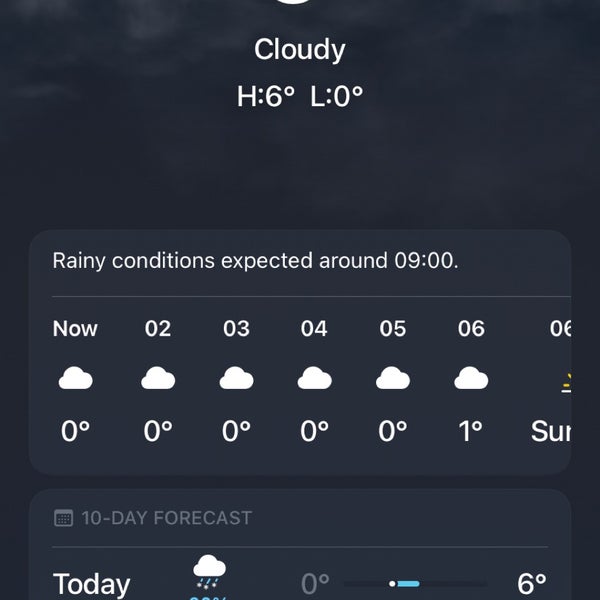This screenshot captures a partial view of a weather app on a smartphone screen. The overall theme of the app has a dark, cloudy background. Centrally located at the top, white text displays "Cloudy" along with the high and low temperatures of the day, indicated as "High: 60°F" and "Low: 0°F" using the abbreviations "H" and "L" respectively. 

Below this information, a dark gray box features lighter gray text that reads, "Rainy conditions expected around 0900." Underneath, the current weather conditions are presented in a vertical format, each accompanied by a cloud icon:

- 0000: 0°F (cloudy)
- 0100: 0°F (cloudy)
- 0200: 0°F (cloudy)
- 0300: 0°F (cloudy)
- 0400: 0°F (cloudy)
- 0500: 0°F (cloudy)
- 0600: 1°F (cloudy)

Returning to the "now" segment, there is a cloud icon followed by a temperature of 0°F. The cloud icon and temperature format are consistent throughout.

At the bottom of the display, there is a section featuring a calendar icon labeled with a "10-Day Forecast." This area currently highlights "Today," showing a cloud icon indicating snow due to the freezing temperature of 0°F. Following this, a blue line highlights a forecast of 6°F alongside the continuous snowy icon.

The detailed layout and iconography clearly depict the ongoing cold, cloudy, and snowy weather conditions.